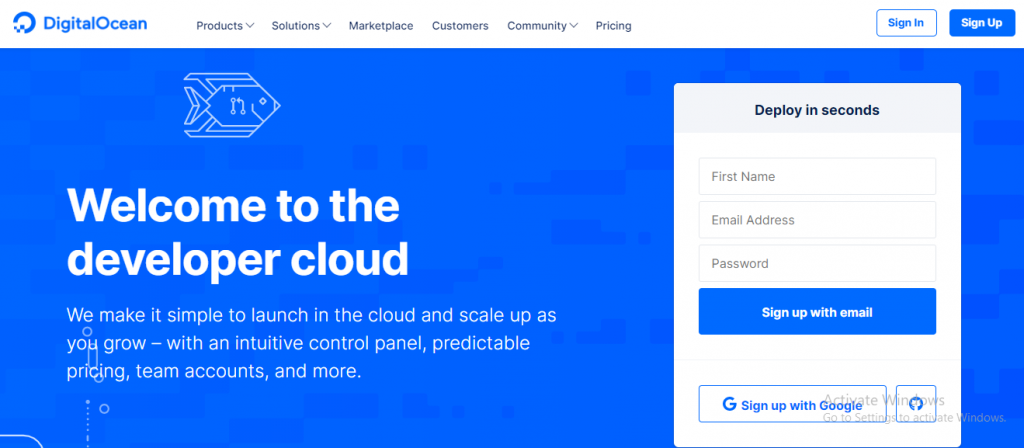The image is a promotional shot for Digital Ocean, prominently featuring their trademark elements. At the top, "Digital Ocean" is displayed in bold, bright blue text alongside their distinctive emblem: a wide, open circle with a segment from nine o'clock to six o'clock composed of small check marks, giving the 'O' an incomplete appearance.

The main navigation bar includes options such as Product, Solutions, Marketplace, Customers, Community, and Pricing. Just below and slightly left of center, there's a charming sketch of a fish adding a playful touch to the design.

Dominating the center of the image, in large, bold white text, is the welcoming message: "Welcome to the Developer Cloud." The message beneath simplifies their value proposition: "We make it simple to launch in the cloud and scale up as you grow with an intuitive control panel, predictable pricing, team accounts, and more."

On the right side of the image, a pop-up box encourages users to "Deploy in seconds." It asks for the user's first name, email address, and password, offering the option to sign up either via email or Google. The entire layout, characterized by vivid blue backgrounds and clean white text, conveys a sense of clarity and reliability.